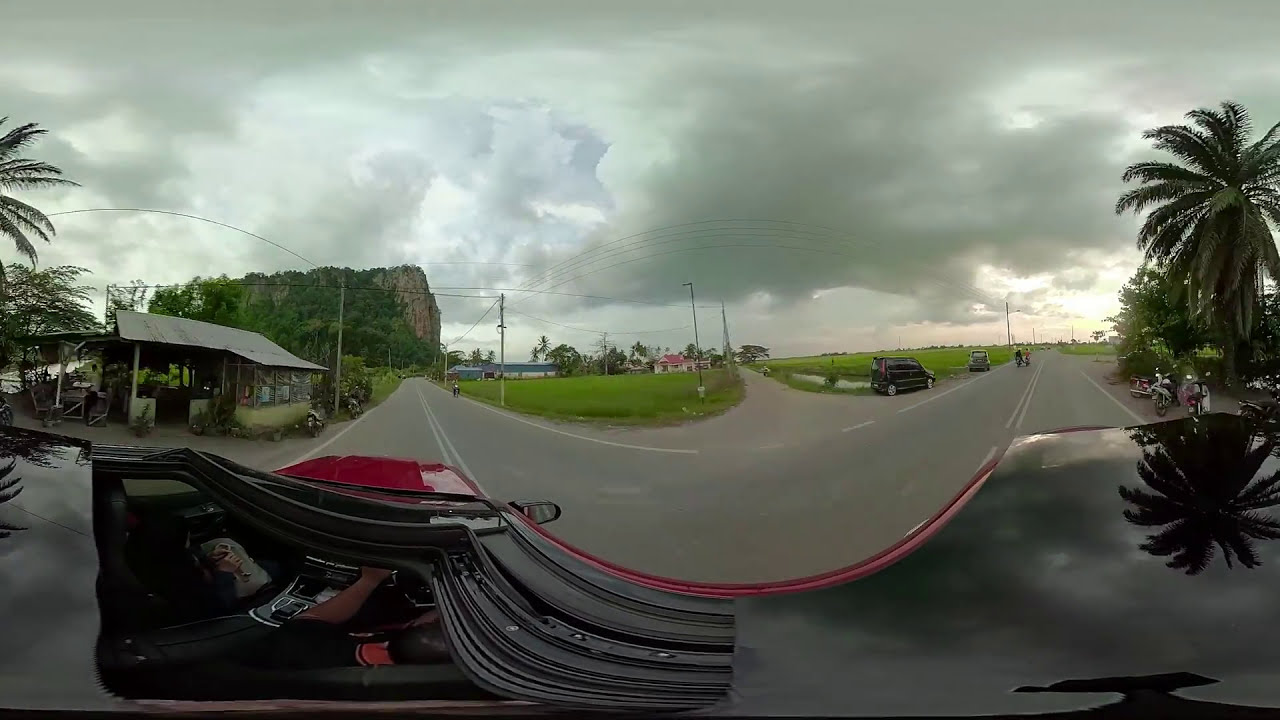This panoramic 360-degree outdoor image captures a heavily distorted scene from within a vehicle. At the bottom, part of the vehicle's black hood with red accents is visible. Inside, you can also see the car's console and the driver. The road ahead splits, linking two directions of the highway into a continuous loop that straightens toward the middle of the image. To the front right, one road makes a sharp curve, while another appears as a smaller path without lines.

On the left side, several parked scooters line the road near an old hut or possibly an outdoor fast-food stand with a metal roof on posts. This building, reminiscent of an old-fashioned burger place, adds to the scene's nostalgic feel. In the distance, someone rides a scooter towards the viewer. Palm trees and a variety of other trees frame both sides of the highway, supplementing the background filled with cloudy, overcast skies and looming thunderheads. Additional vehicles, including SUVs and motorcycles, are also scattered along the roadside, contributing to the bustling yet distorted ambiance.